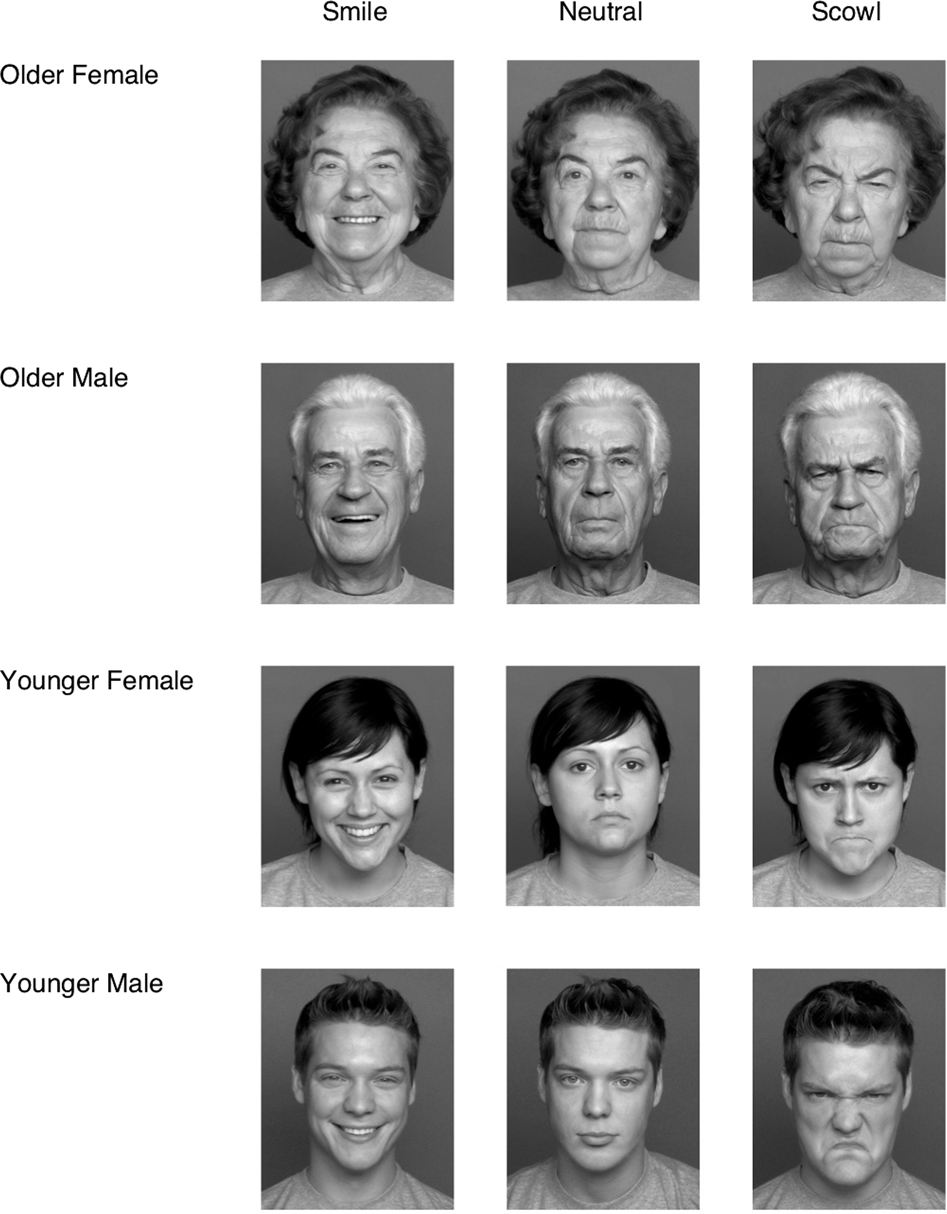The image consists of a grid of 12 black and white photos organized into four rows and three columns. The rows feature four individuals—an older female, an older male, a younger female, and a younger male—from top to bottom. Each individual is depicted three times across the columns, showcasing different facial expressions from left to right: smiling, neutral, and scowling. At the top of each column, labels indicate the expression ("Smile," "Neutral," "Scowl"), while labels at the beginning of each row identify the individuals categorically ("Older Female," "Older Male," "Younger Female," "Younger Male"). All expressions appear genuine, with a notable deviation where the younger male shows a subtly happy demeanor even in his neutral photo. The artistic coherence of the black and white photos enhances the overall impact, making the composition visually striking and emotive.